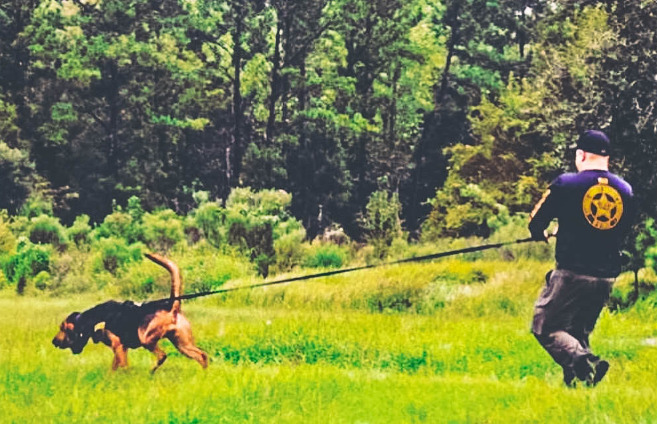The image is an outdoor daylight photograph of a police officer and a search dog in action. Taken from behind, the scene captures the pair in a grassy field with tall, yellowish-green grass and patches of dirt, shrubs, and scattered greenery. The dog, which appears to be a bloodhound with brown fur, big floppy ears, and a long tail, is on the left. It's wearing a substantial harness and a vest connected to a long black leash held by the officer. The dog is straining forward with its nose close to the ground, clearly in search mode.

To the right, the police officer has a stocky build and is wearing a black baseball cap, a blue long-sleeved shirt with a sheriff's star badge in gold on the back, and dark cargo pants. The background is a dense wall of forest vegetation and tall trees, creating a natural, somewhat wild setting. The overall image has an overexposed appearance, suggesting it may have been originally taken on film and later scanned digitally.